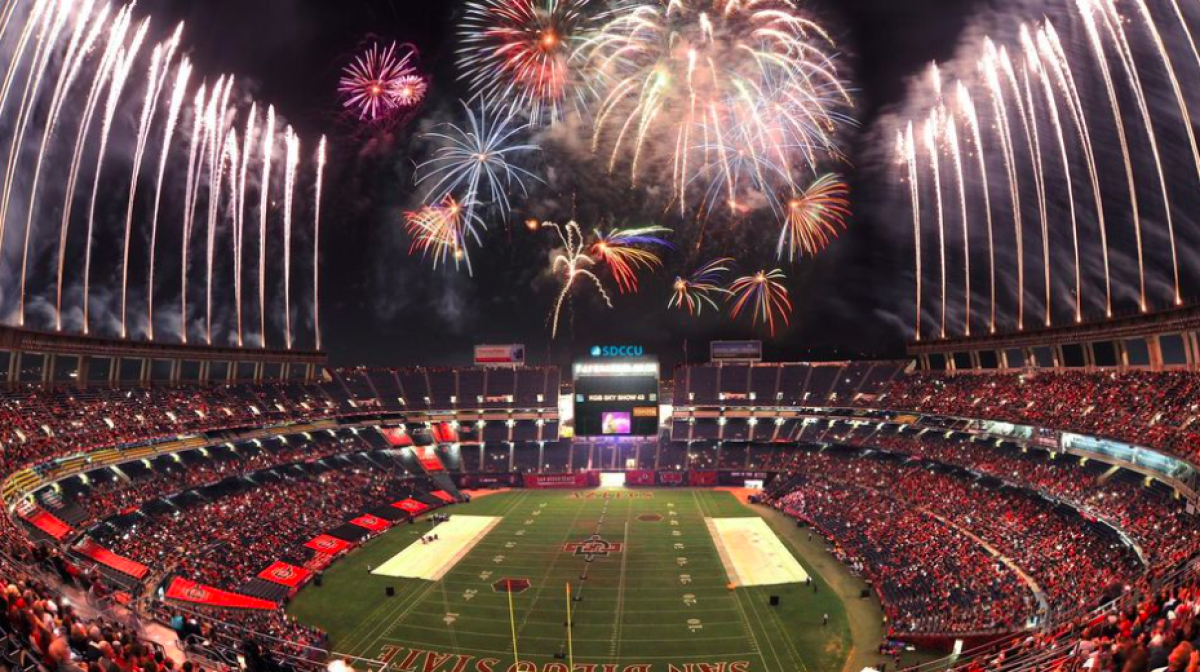The image depicts a grand outdoor stadium, unmistakably a football stadium, brimming with energy and color. The expansive green field is central, bordered by vividly yellow field goalposts, and marked at the bottom with “San Diego State” in the end zone. The stadium, towering with nearly four levels of seating, is packed to capacity, creating a sea of red as whether through the crowd’s attire or possibly the color of the seats themselves. The scene is set at night, with the upper half of the image enshrouded in a dark sky. A magnificent fireworks display dominates the background, centered at the top, with additional sparkler-like illuminations or potentially water features flanking each side at the stadium's apex. The festive atmosphere is underscored by bright lights and spectators on the sidelines, appearing tan with occasional white patches, encapsulating a moment of celebration without any players visibly on the field.